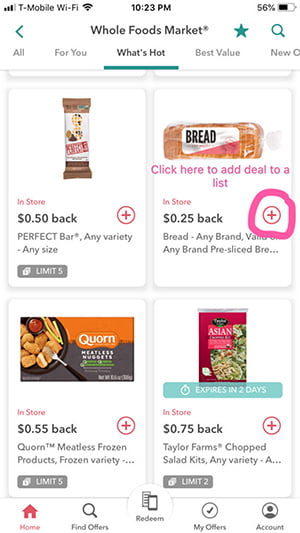This image is a photograph of a phone screen displaying an advertisement from Whole Foods, captured at 10:23 p.m. on a T-Mobile device. The main heading of the ad reads "All For You" and features sections titled "What's Hot," "Best Value," and "New Product." Four promotional offers are highlighted:

1. **Perfect Bar**: Any variety and size of this protein bar qualifies for a $0.50 cashback reward. This offer is available in-store only and has a limit of five bars. To take advantage of this offer, one would need to click on the round pink circle with the plus sign.

2. **Sliced Bread**: Any brand of pre-sliced bread qualifies for a $0.25 cashback reward. The offer is visually indicated as active by a pink circle outlined with a pink marker.

3. **Quorn Meatless Frozen Products**: These plant-based meat alternatives offer $0.55 cashback per item, with a limit of five items. To redeem, click the pink circle with the plus sign beside the product listing.

4. **Taylor Farms Salad Kits**: This offer includes any variety of Taylor Farms salad kits, with an example shown featuring an Asian salad kit. The offer, which expires in two days, provides $0.75 cashback per kit and has a limit of two. Redemption also requires clicking the pink circle with the plus sign.

Each product offer is accompanied by detailed conditions including cashback amounts, product limits, and redemption instructions.